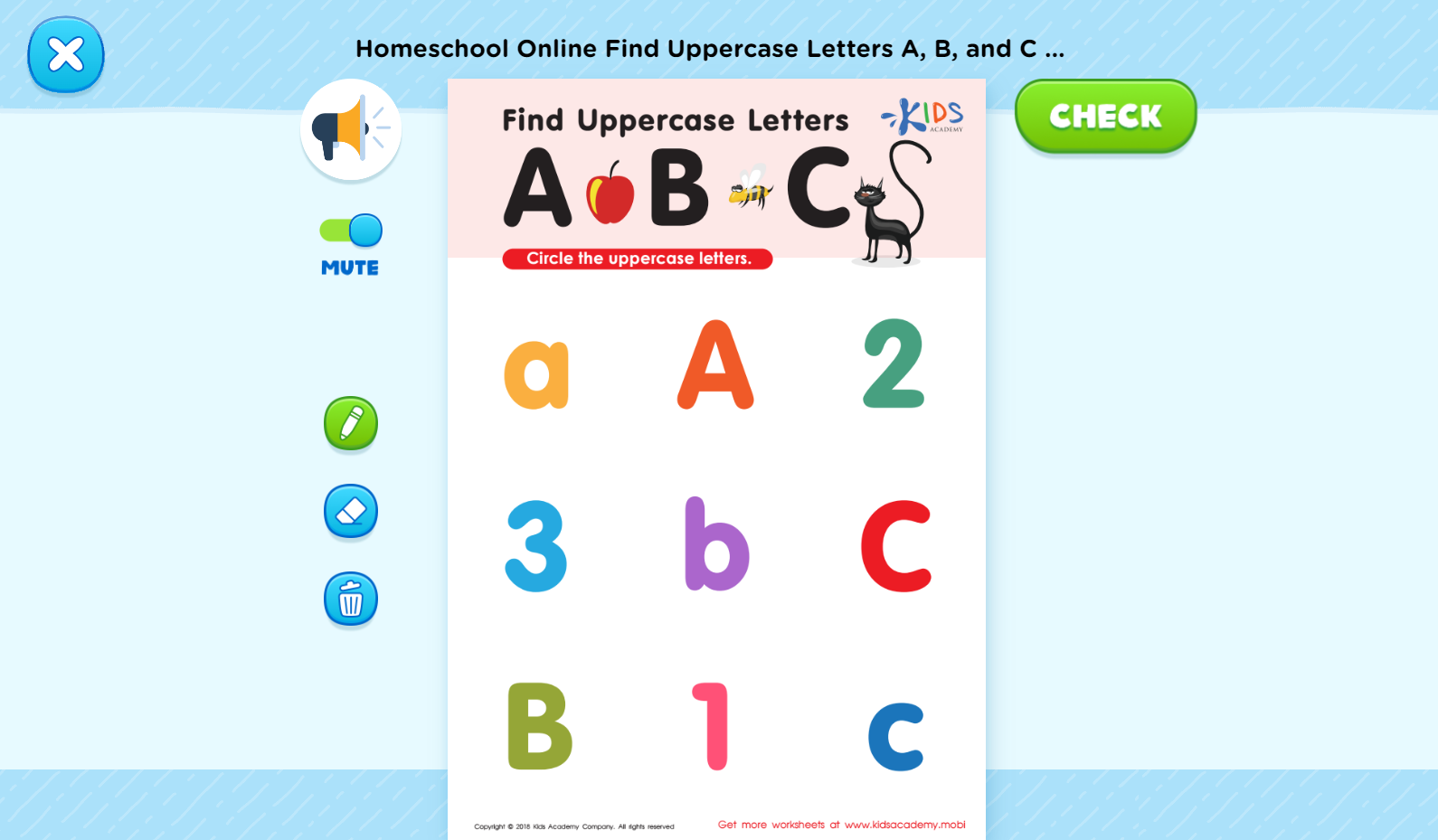This is an image of an educational website designed to teach children their ABCs and 1, 2, 3s. The background of the webpage features a light blue color, with darker blue rectangular sections at both the top and bottom. In the top left corner, there is a clickable white 'X' inside a blue circle, allowing the user to close the page. Centrally located at the top, bold black text reads "Homeschool Online: Find Uppercase Letters A, B, and C...".

Directly beneath this heading, on the upper left side, you'll find a speaker icon which can be clicked to hear the letters aloud. Next to it, a mute slider is visibly turned on. Further down, there are icons for a pen, an eraser, and a trash can, likely used for interactive activities. The main instruction section in the middle of the page states, "Circle the Uppercase Letters," accompanied by a mix of uppercase letters, numbers, and lowercase letters for the child to identify and circle the correct uppercase ones. In the upper right corner, there is a green check button, presumably for submitting answers or verifying them.